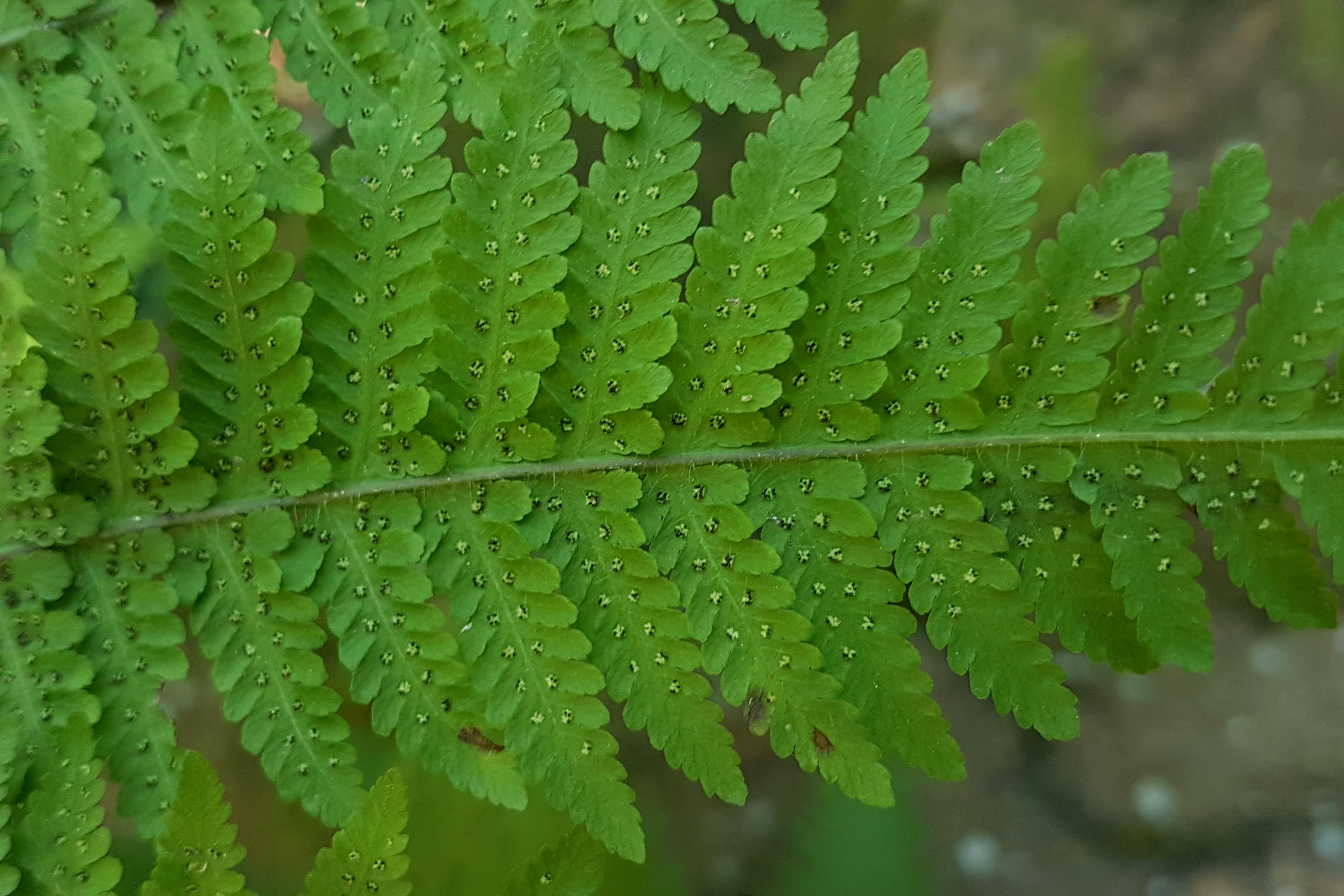This close-up image captures a vibrant green fern leaf in intricate detail. The fern stretches horizontally across the frame, with a dark green central stem running through the middle. From this central stem, multiple smaller leaflets, each measuring about two to three inches in length, radiate outwards in a symmetrical pattern. These leaflets are arranged diagonally and horizontally, creating a lush, layered appearance. The leaflets are a bright shade of green, adorned with tiny, golden-hued dots that might resemble water droplets or pollen, evenly distributed along each leaflet. These golden specks add a delicate, almost sparkling quality to the leaf’s surface. The leaf tapers into a pointed tip, emphasizing its elegant, elongated form. The background is blurred, giving a sense of being outdoors and allowing the detailed texture of the fern leaf to be the focal point.